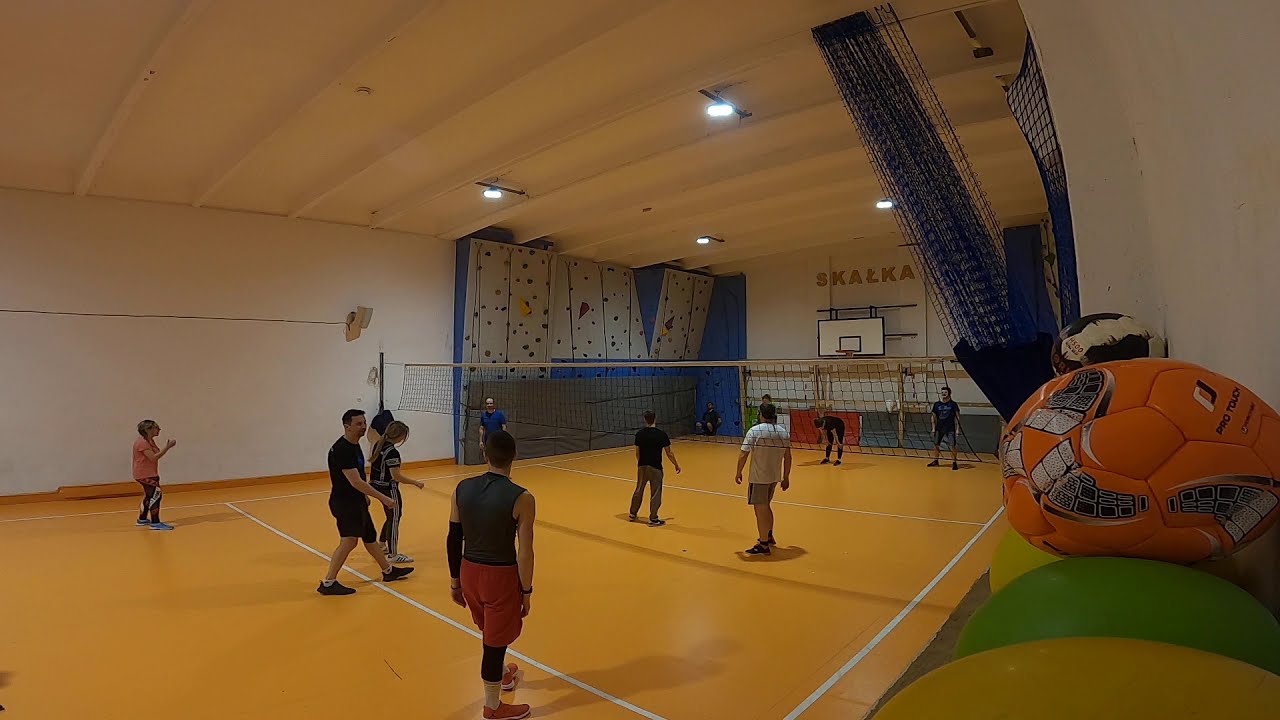This image is a detailed color photograph of an indoor volleyball game taking place in a multi-purpose gymnasium. The court, situated inside a spacious building with high ceilings, appears to be a repurposed basketball court with a net set up at mid-court. On the court closest to the camera, there are about eight players, predominantly men, with a mix of genders, dressed in gym attire such as shorts and t-shirts. On the opposite side of the net, there are approximately four to five players and one person leaning against a blue wall.

The gym floor is a bright orange color with various lines marking the volleyball and basketball boundaries. In the background, there is a white climbing wall with numerous handholds, indicating this gym also supports rock climbing activities. Off to the right side of the image, there is a blue net suspended from the ceiling and several multi-colored balls, including an orange soccer ball and yellow and green balls, piled up in the foreground. Additionally, a basketball hoop is visible further to the right, suggesting the versatile use of the space. The word "Shalka" or a variation of it with a unique character resembling a Russian "L" with a dash is noted on the floor, hinting at possibly international or cultural influences within the gym.